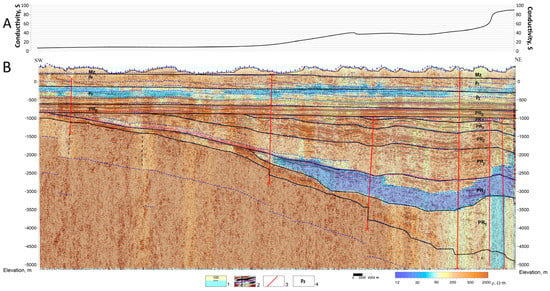The image is a detailed diagram depicting a cross-section of land with distinct layers and a color spectrum key at the bottom. The primary background of the diagram is brown, representing the earth or soil. A prominent rectangle dominates the center, featuring rows and curved lines in dark blue. These blue lines appear to signify different strata or possibly water or mineral deposits within the ground. On the left and right sides of the rectangle, numerical values ranging from 0 to 150 are written along the y-axis, albeit in small and hard-to-read font. In the top left corner of the image, the letters "A" and "B" mark the diagram's reference points. 

A color spectrum key at the bottom transitions from dark blue to lighter blue, then yellow, orange, and red, indicating varying levels of data, potentially conductivity or mineral content. Additionally, the word "conductivity" appears on the right side, written sideways. The entire diagram has a patchwork of hues, including blue, tan, and red, with various lines and markings. Purple lines resembling stitching traverse the image, adding texture or denoting specific measurements. The overall appearance suggests that the diagram is a detailed representation of subsurface features, possibly used for geological or hydrological analysis.